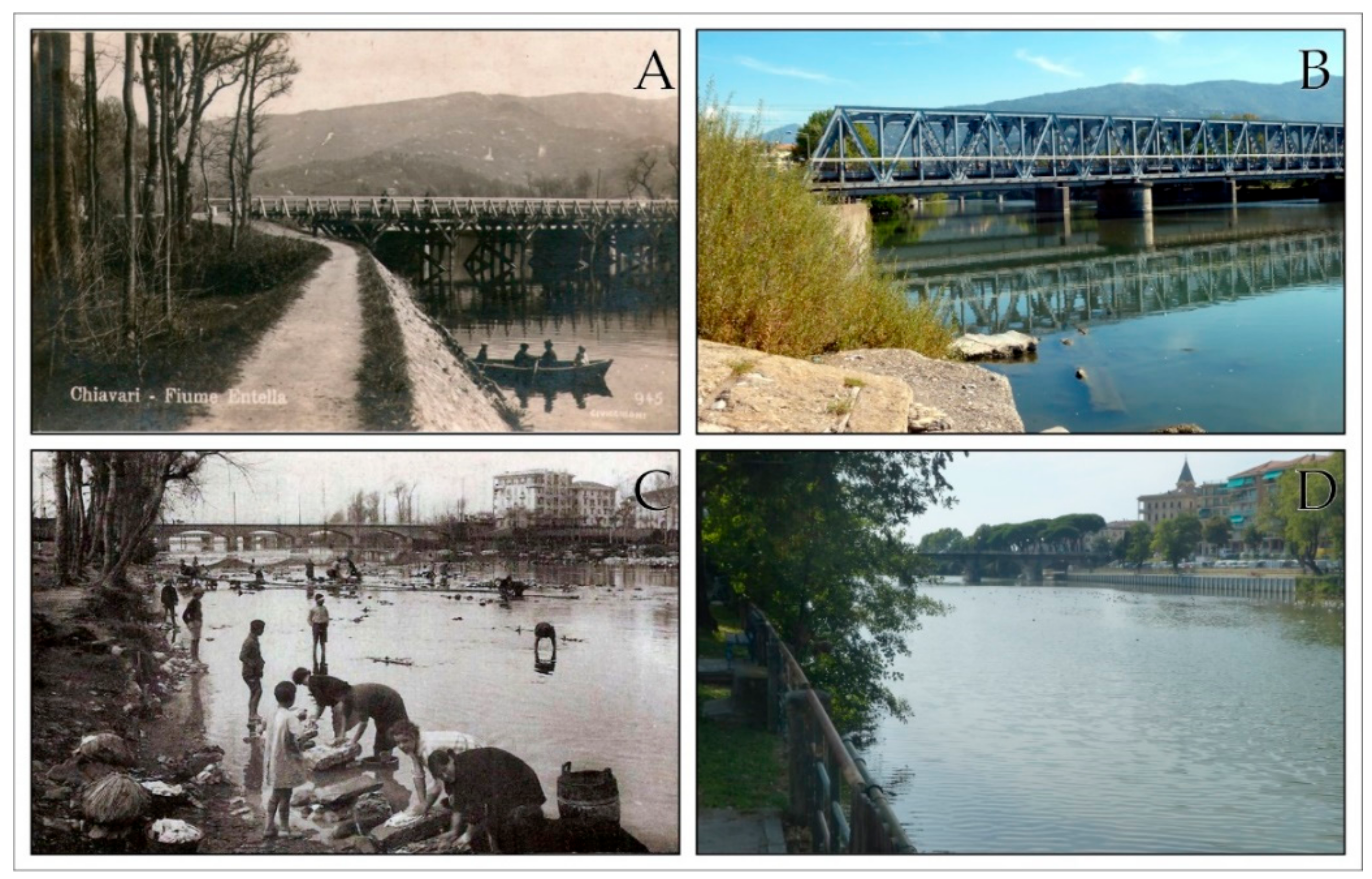This image is a compilation of four distinct photographs, each labeled A, B, C, and D in the upper right corner of each section. 

In the top left (Image A), the photograph, which has a sepia tone, depicts a historical scene of a bridge named "Shafari Fiume Antela." This image showcases a waterway with four people in a boat, surrounded by barren, tall, thin trees and a pathway. The bridge itself is slightly less detailed, adding to its antique feel.

The top right photograph (Image B) presents a modern contrast to Image A. This colored photo features a blue, contemporary bridge with a triangular pattern, visible across the clear blue water. In the foreground, a rock face adorned with a green bush is noticeable, adding a touch of nature to the scene.

In the bottom left (Image C), another black and white photograph highlights a polluted river shoreline where individuals are seen washing and picking things up. The bridge in the background features large archways, emphasizing the more industrial and unclean aspect of this scene.

The bottom right photograph (Image D) offers a contemporary view similar to Image B. This colored photograph displays clear blue water with a green tree on the left. In the distance, a modern flat bridge is visible, contributing to the serene and clean aesthetic of this more recent image.

Together, these four photographs illustrate a contrast between historical and modern scenes, as well as varying environmental conditions surrounding bridges.